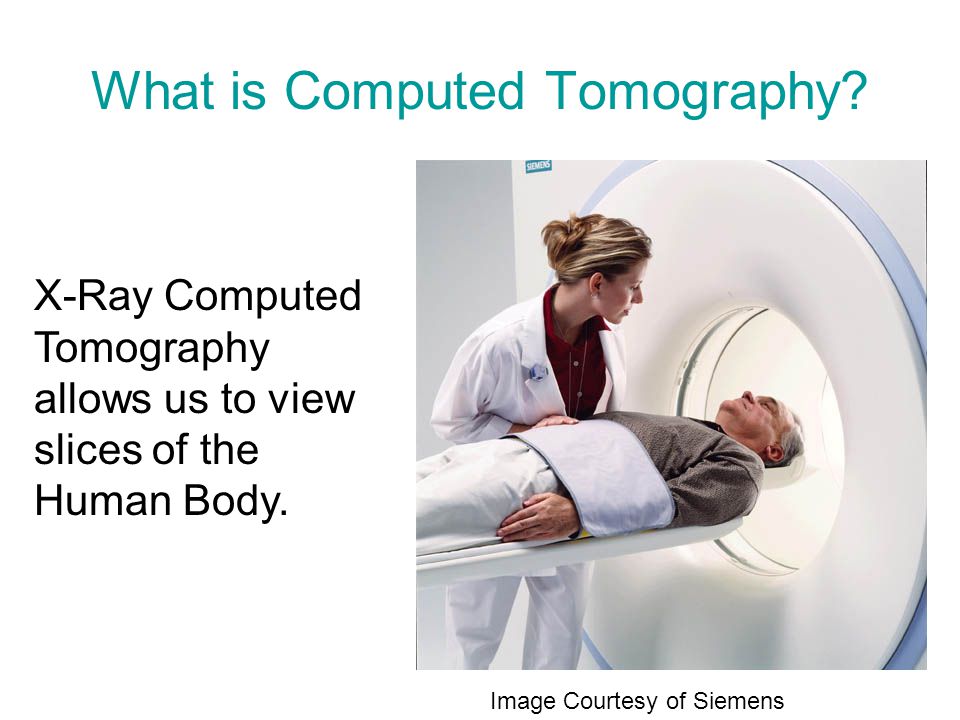This image features a medical setting with a white background, making the green and black text prominent. At the top, in green font, the text reads, "What is computed tomography?" To the left, in larger black font, it states, "X-ray computed tomography allows us to view slices of the human body. Image courtesy of Siemens." On the right side of the image, an elderly white gentleman with white-grayish hair, wearing a brown shirt and white pants, is being inserted into an MRI machine. His midsection is covered with some cloth, and his arms are held to his sides. Assisting him is a woman in a white lab coat, white pants, and a red button-down shirt, with her blonde hair pulled back. The overall scene appears to be part of a medical PowerPoint slide illustrating the concept of computed tomography.